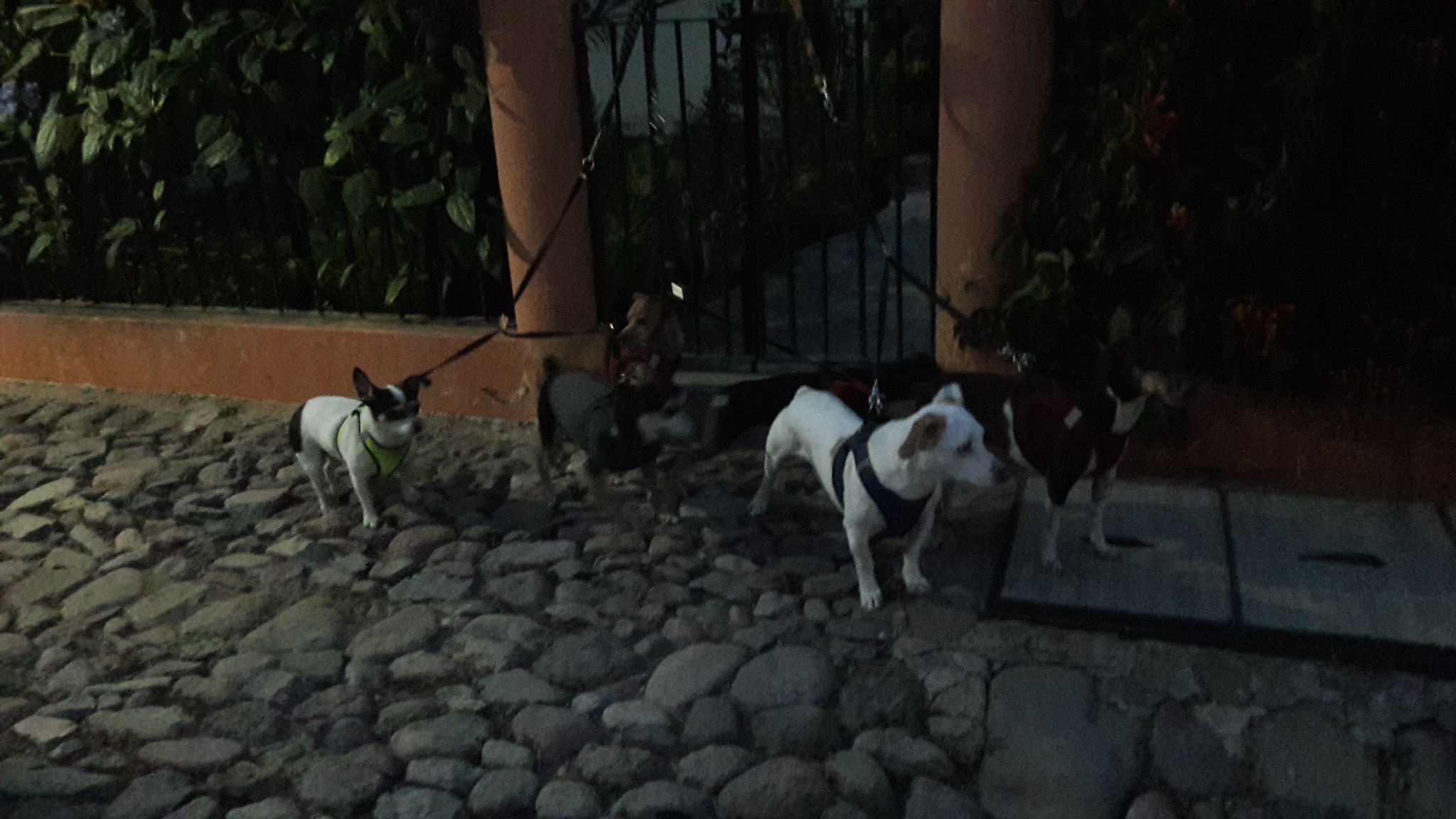In this candid outdoor photograph, likely taken on a phone, six small to medium-sized dogs of various mixed breeds and colors are tied to a gate in front of a home with stone pavement. The dogs, standing on cobblestones with a hedge and gate in the background, are all well-behaved and seem to be waiting patiently for their owner, ready for a walk. Frontmost is a small white dog with a black nose and brown ears, wearing a bluish harness. Next to it, a small lion chihuahua is distinguishable by its lime green vest and harness. The dogs are all facing the same direction, towards the right, enhancing the impression of anticipation and coordination.